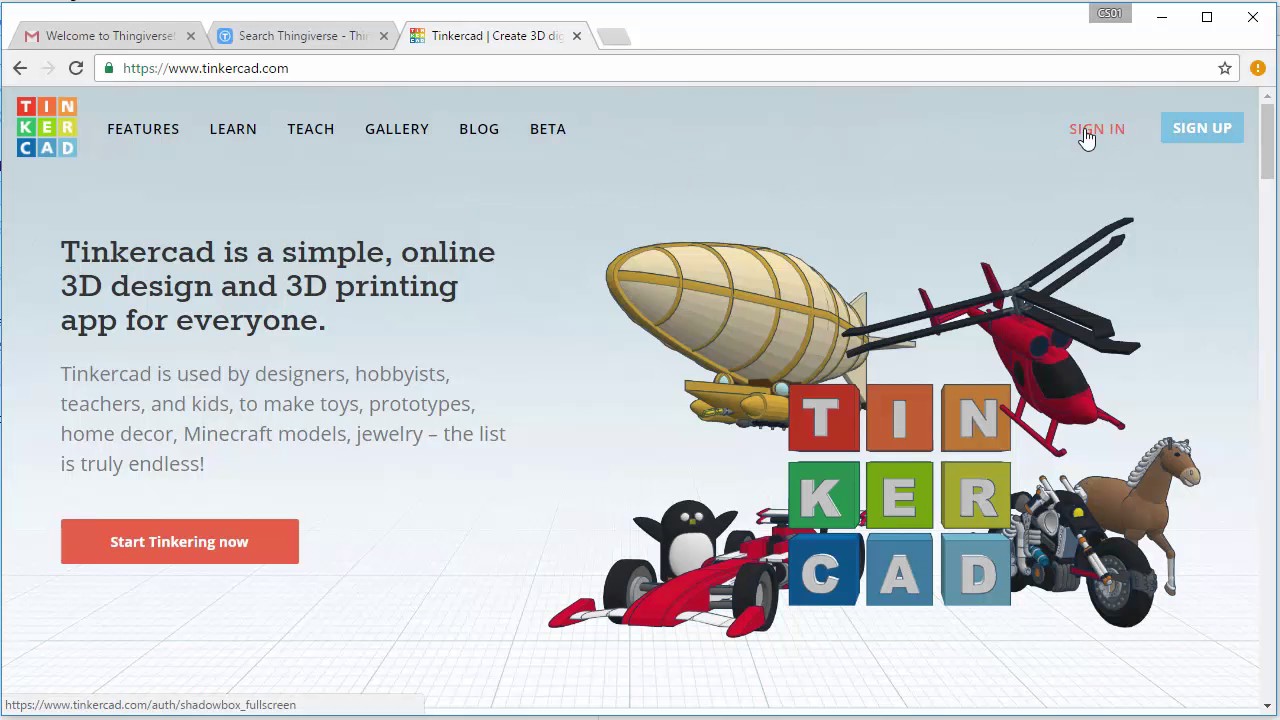The image showcases the front page of the Tinkercad app, a user-friendly online platform for 3D design and 3D printing. At the top left corner, the Tinkercad logo is prominently displayed, featuring a vibrant, rainbow-colored gradient that transitions from red to orange for "TIN," green to yellow for "KER," and blue to light blue for "CAD." The background mimics a 3D horizon, making the logo appear as if it is integrated within the 3D space, resembling the environment where users create their designs.

Navigation options are clearly laid out at the top, including "Features," "Learn," "Teach," "Gallery," "Blog," and "Beta." A hand icon hovers over the "Sign In" button, which is situated to the left of the "Sign Up" option. This layout encourages new users to get started and existing users to jump back into their work seamlessly. The caption emphasizes Tinkercad's mission to make 3D design accessible to everyone, encouraging users to "Start tinkering now." The overall design of the page is clean and inviting, perfectly suited for beginners and experienced designers alike.